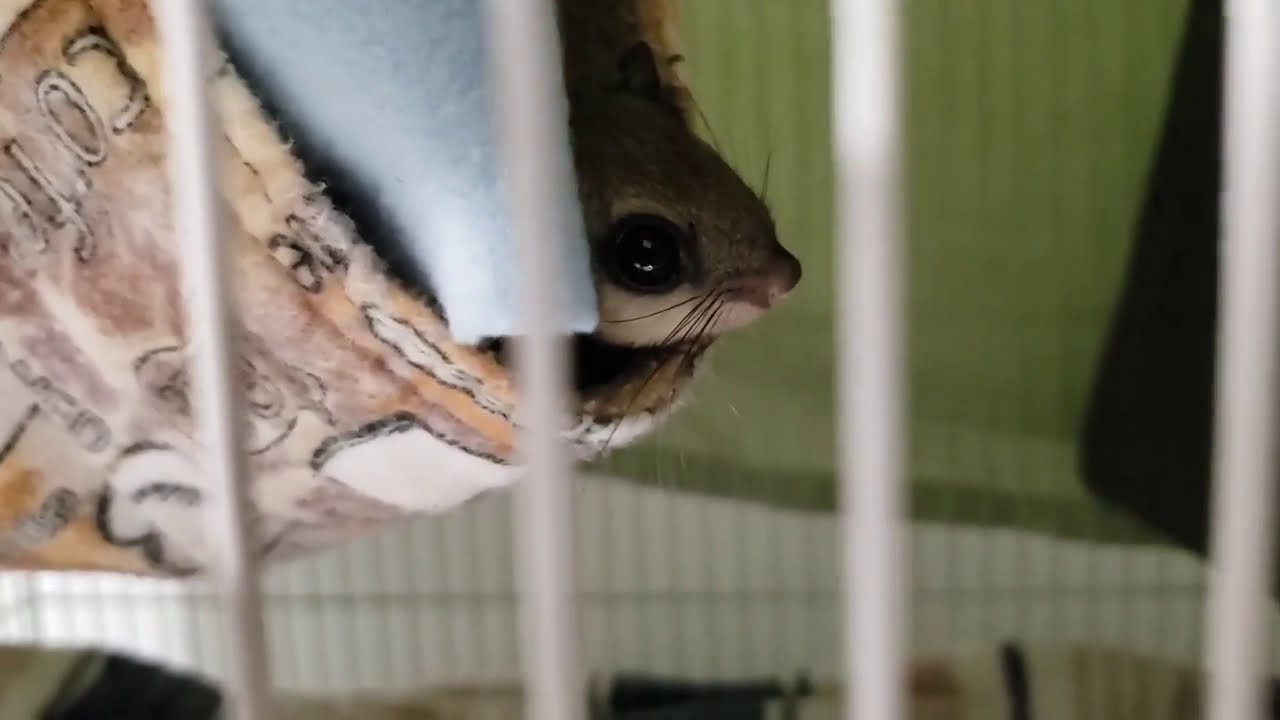The close-up photograph captures the view from just outside a small animal's cage, displaying four circular, vertically-aligned bars at the foreground. Enveloped in a cozy, U-shaped fabric cradle, a small rodent — likely a mouse or a gerbil — peeks out, revealing only its head adorned with a large black eye. The animal's profile showcases its black whiskers, small reddish-brown nose, light brown fur, and a touch of white fur beneath its eye, along with a faint glimpse of an ear atop its head. The fabric cradle, which may be part of a jacket sleeve or a specially designed pet bed, is primarily brown and contains hints of blue fabric patterned with some letters. Behind the animal, a green wall and a white baseboard are visible, with a towel draped over the cage, suggesting the setting is a comfortable pet room.